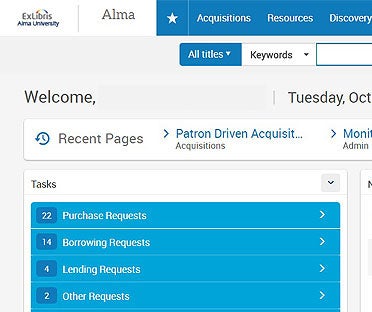A screenshot from the Ex Libris Alma Library Management System at Alma University, highlighting the interface on Tuesday, October 22nd. The image features the search functionality at the top with options like "All Titles" and "Keywords" in the search box. 

On the left side, under the "Recent Pages" section, there are several patron-driven acquisition requests listed with corresponding arrows indicating their categories: 14 purchase requests, 4 borrowing requests, 2 lending requests, and other requests.

In the top bar, navigation options such as "Resources," "Discovery," and administrative tasks are visible, and there's a dropdown menu for additional actions next to the "M" icon. There is also a date and time display including a welcome message and an indication of the current status within the library system.